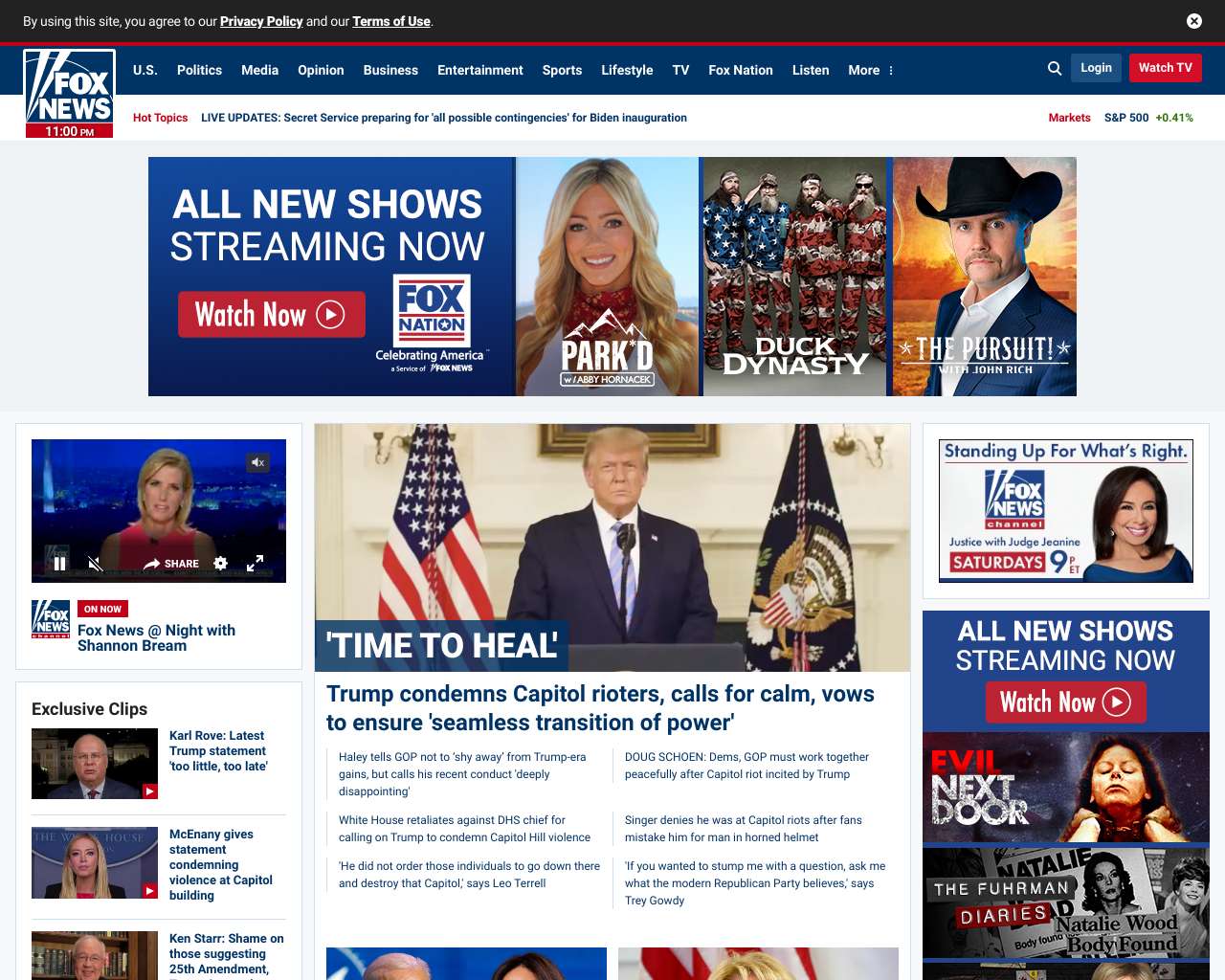The image captures the Fox News website at 11:00 p.m. The top section of the website features a blue header with navigation links highlighted in white font, including U.S., Politics, Media, Opinion, Business, Entertainment, Sports, Lifestyle, TV, Fox Nation, Listen, and More. Additionally, options for login and watching TV are available.

Beneath the header, the site transitions to a white canvas showcasing a headline under the section labeled "Hot Topics" and "Live Updates." The headline reads, "Secret Service preparing for all possible contingencies for Biden inauguration."

Below this, there are three images representing different shows currently streaming on Fox Nation:

1. "Parked" - featuring a female.
2. "Duck Dynasty" - featuring four individuals.
3. "The Pursuit" - featuring a male in a blue suit and black cowboy hat.

Accompanying this is a call to action: "All new shows streaming now. Watch now, Fox Nation."

Further down, a collage of clickable tiles is displayed. The left column features a news broadcast segment titled "Fox News Night with Shannon Graham," followed by a section called "Exclusive Clips" with three featured clips:

1. Karl Rove discussing the latest Trump statement, titled "Too little, too late."
2. Kayleigh McEnany giving a statement condemning violence at the Capitol Building.
3. Ken Starr criticizing suggestions of invoking the 25th Amendment, though the full title is cut off.

In the center of the page, there's a prominent image of President Trump, accompanied by the message "Time to heal." Below it, a headline reads, "Trump condemns Capitol rioters, calls for calm, vows to ensure seamless transition of power," followed by segments with smaller text discussing:

- Haley urging the GOP not to shy away from Trump-era gains, while also expressing disappointment in his recent conduct.
- The White House retaliating against the DHS chief for calling on Trump to condemn Capitol violence.
- Leo Terrell stating that Trump did not order the violence at the Capitol.

Several other texts are present but are too blurred to read clearly.

On the right side of the screen, an advertisement for "Justice with Judge Jeanine" broadcasts Saturdays at 9 p.m. Eastern Time. A clickable link underneath promotes new shows streaming now, accompanied by a "Watch Now" button. Below this, the show "In Town, Evil Next Door" is mentioned, followed by "The F.U.H.R.M.A.N. Diaries: Natalie Wood, Body Found."